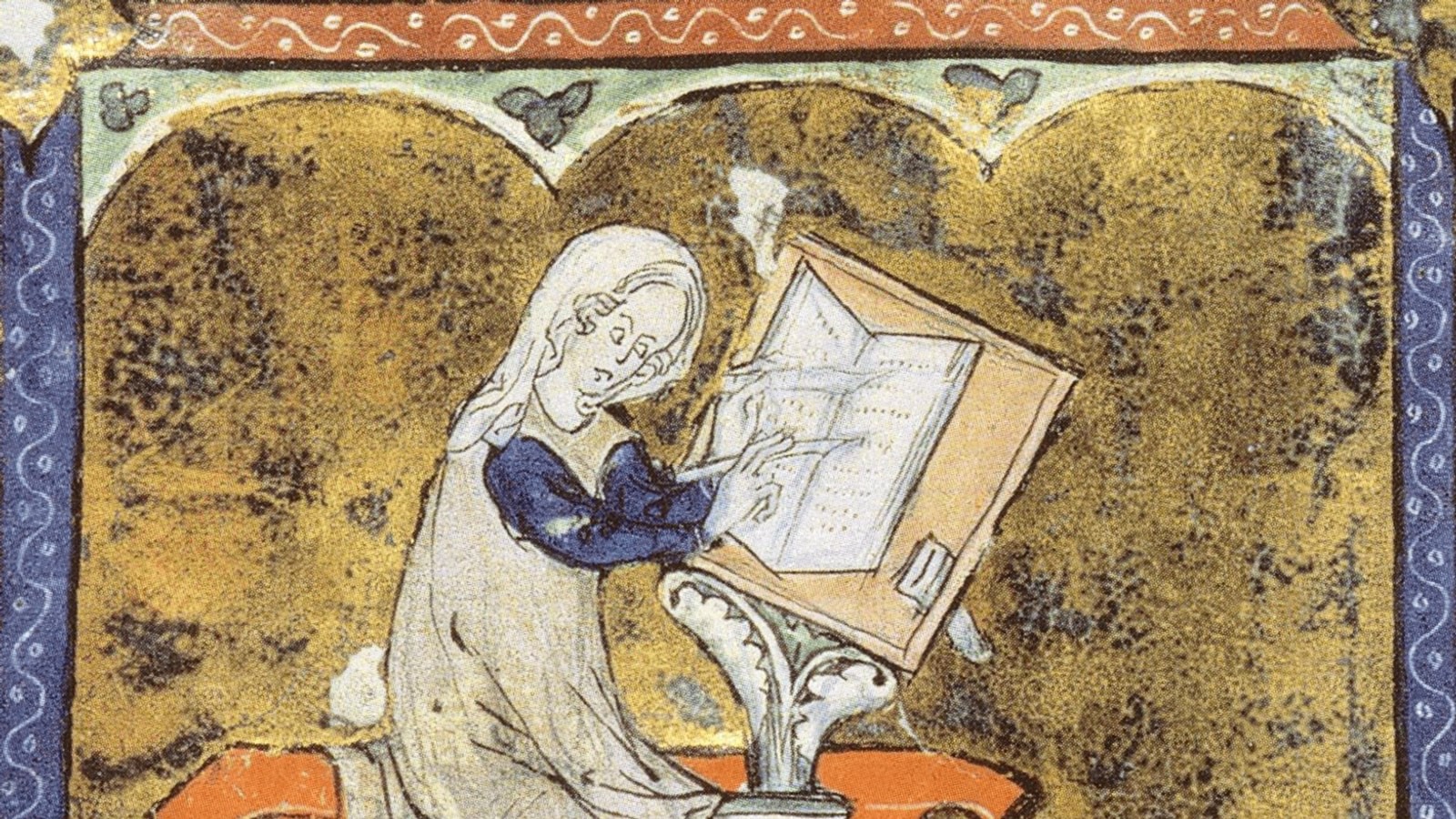The image is a detailed illustration or painting with a rich, dark tan background framed by an intricate blue border adorned with white swirls and circular patterns. Central to the image is a young woman, possibly a nun, seated on an orange-brown wooden bench. She is wearing a long sleeveless gown over a blue long-sleeve shirt, and her appearance suggests she might be from the Renaissance period. The woman has white hair and is deeply engrossed in her work, holding a pen or pencil, poised to write in an open book or notebook. In front of her is a stand, resembling a music stand, with sheets that appear to contain music notes or writing material. Her focused demeanor suggests she is either writing or studying diligently.